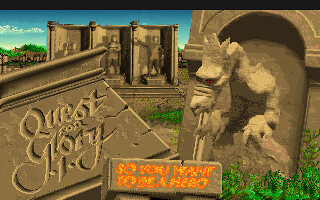This is an image that looks like a screenshot of a retro video game, characterized by its pixelated graphics. Prominently featured in the front left corner is a fallen wooden or stone carved structure that reads "Quest for Glory." Below it, another stone bears the title "So You Want to Be a Hero" in bright yellow with red outlines. Dominating the foreground is a three-dimensional dragon, its red eyes glowing menacingly as it appears to emerge from the stone. The dragon's head and arms are visible while the rest of its body is embedded within the structure. Scattered throughout the scene is green grass, adding a touch of nature to the setting. In the background, under a clear blue sky capped with a thin black line, stand three additional stone structures, each housing statues. The scene is intricately detailed, blending elements of ancient carvings with classic video game imagery.